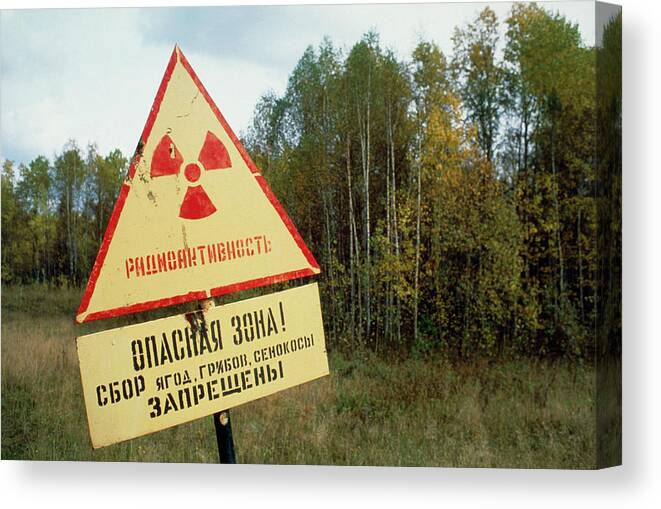This photograph captures a warning sign located in a field filled with overgrown weeds and tall grass, exhibiting shades of green and brown. The signpost supports two signs: the top one is a slightly rusted, yellow triangle with a red border featuring a radioactive symbol—a small red circle with three fanned-out sections radiating from it. Below the symbol is red text, presumably in Russian. The second sign, rectangular and yellow, is situated directly beneath the triangular one, displaying additional information in black Russian text. The scene is set against a backdrop of a tree line, comprising mostly slender trees with white bark. The leaves exhibit various hues, predominantly green, but also some gold and brown. To the left of the image, the sky is visible, filled with blue shades and scattered white clouds.